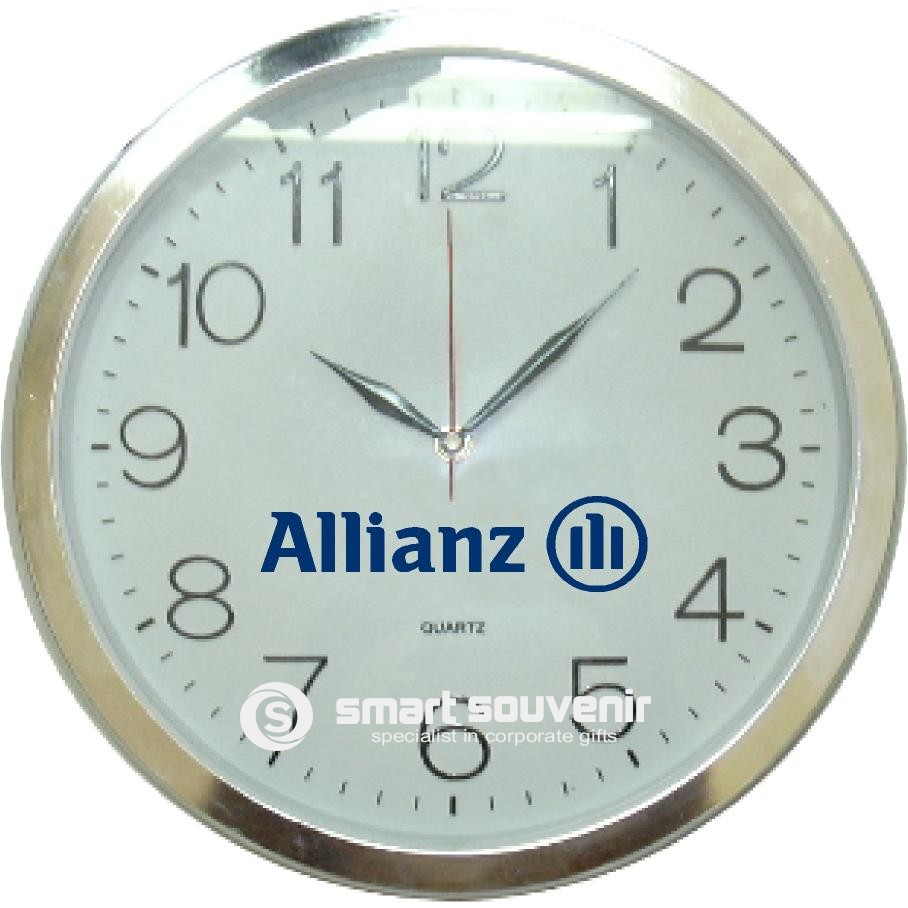This image depicts a close-up view of a large, round, silver clock with a very simple and basic design. Dominating the entire frame, the clock has a shiny, metallic silver bezel and a light gray face. The background around the clock is purely white, adding to the stark simplicity of the image. The numbers on the clock are large, easy-to-read, and have a silvery hue, clearly indicating the hours in a standard 12-hour format. The slender, silver hour and minute hands contrast with the bright red, needle-like second hand. The hour hand points to 10, the minute hand rests between the 1 and the 2, and the second hand is precisely at the 12, indicating the time as 10:08. 

At the center of the clock face, below the hands, is the text "Allianz" in blue, the name of the insurance company, accompanied by their logo featuring a circle with three lines. Below this, in smaller text, is the word "Quartz." Further below, a watermark-like imprint reads "Smart Souvenir, Specialist in Corporate Gifts," encircling an "S" within a white circle. The silver frame of the clock reflects light, giving it a polished finish, suggesting it might be a promotional item from a corporate gift catalog.